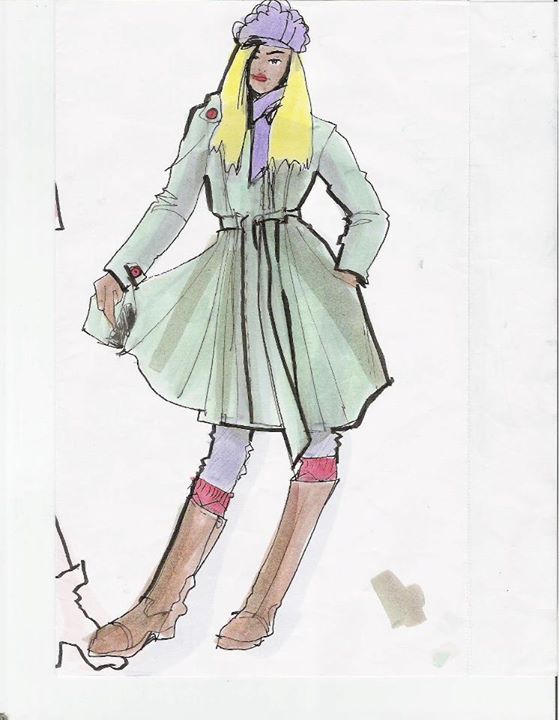This image features a meticulously drawn fashion illustration on a piece of thin paper, likely created using watercolors, ink, and pencil by a fashion designer. The subject of the drawing is a woman with straight, blonde hair who appears to be darker-skinned. She is depicted wearing a modest, mint-green coat that reaches just above her knees and is cinched with a large sash belt that gathers the coat at the waist. The coat is adorned with lapels on the shoulders and red buttons.

Her accessories include a matching light purple hat and scarf. She is also clad in light purple leggings paired with red socks, and tall, knee-high light brown boots. The model is posed with one foot in front of the other, her hip slightly to the side, and her left arm tucked into a pocket, exuding a modern and stylish demeanor.

In the illustration, there is a stain or marking from a brown marker in the bottom right-hand corner of the paper. Additionally, on the bottom left, there appears to be the partial foot of another woman, although it is cut off and not fully visible. This drawing captures the essence of contemporary fashion with its thoughtful details and vibrant color palette.